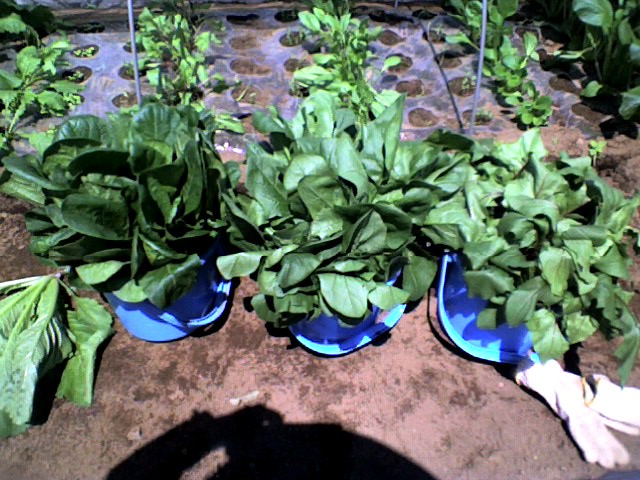This outdoor photograph showcases a meticulously arranged garden scene. Prominently in the foreground, there are three light blue buckets, each brimming with vibrant, dark green plants that resemble large lettuce leaves. The plants in these buckets appear thicker and have longer leaves compared to others in the garden. Surrounding the buckets, the light brown soil is visible, with white gardening gloves lying in the bottom right corner.

The midsection of the image reveals rows of planters embedded in the earth, some containing dense green foliage while others are still empty, exposing the cultivated soil beneath. Interspersed among the planters are sections of plastic sheeting with neatly cut holes, possibly to control weed growth. In the frontmost part of the image, partial shadows suggest the presence of the photographer, adding a human element to this serene garden snapshot. A striking shadow at the top of the image completes this layered, detailed outdoor garden scene.